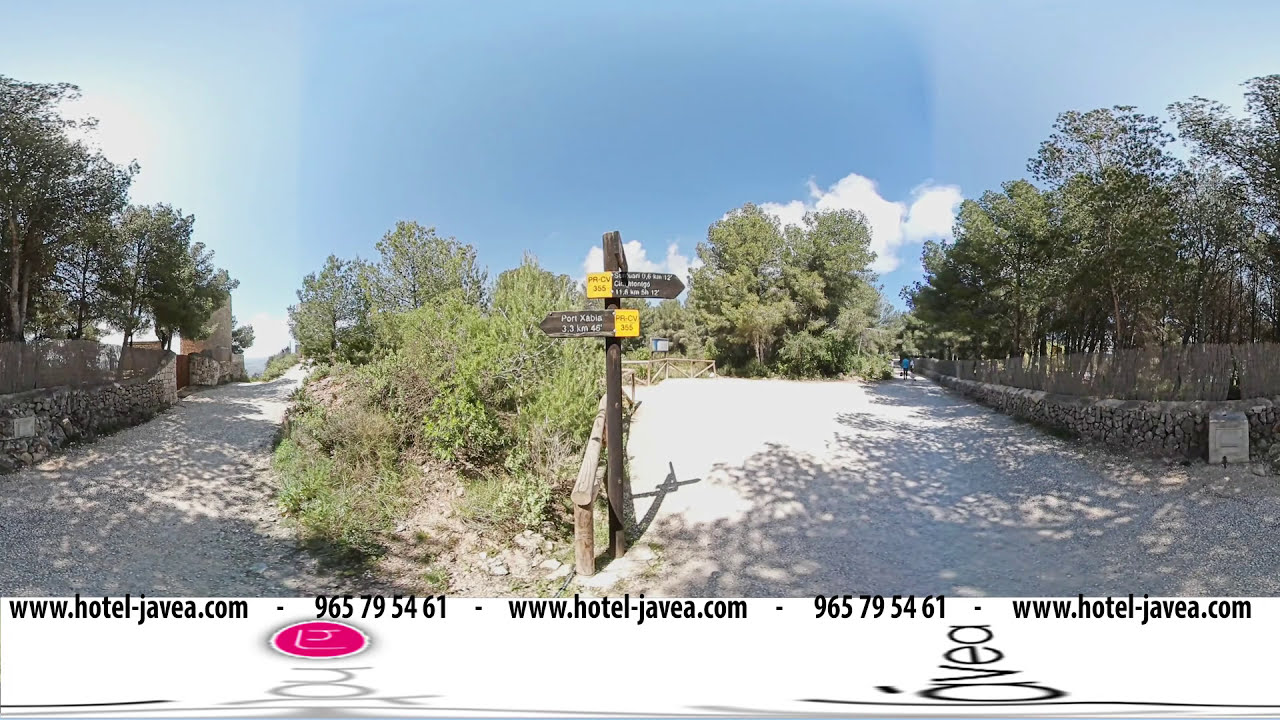The image portrays an outdoor scene of a hotel area, possibly used for advertisement as indicated by the text "hoteljava.com" and logos on the bottom. At the center, there's a prominent dark brown wooden signpost with two arrows: one pointing left and one pointing right. The arrow pointing left displays "Port Xabia, 3.3 kilometers, 46 degrees." In contrast, the arrow pointing right shows "PR CV-365, 11.8 kilometers, 14.12 degrees or 68.12 degrees." 

Surrounding the signpost, there's lush green shrubbery and trees with thin branches mainly at the top. The area features two paths diverging left and right. The left path, edged by a small black fence and bordered with tall trees, seems to lead towards a beach or clearing with blue sky visible in the background. On the right path, more trees and a stone median can be seen, as well as two people walking in the distance. The paths appear to be gravel, flanked by occasional stone walls, adding to the scenic nature of the location.